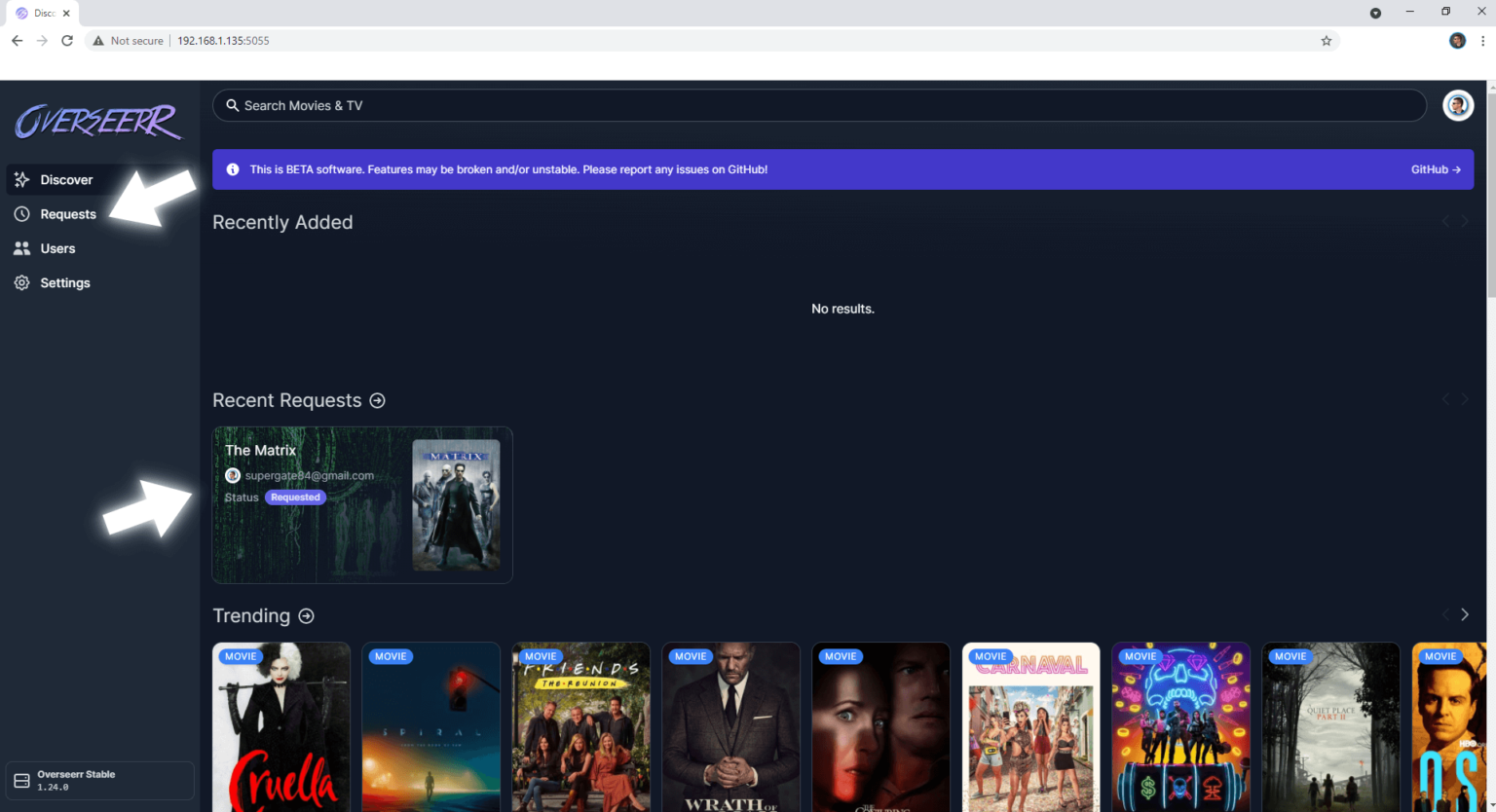**Detailed Image Description:**

At the top of the interface, there is a heading displayed in bold, capital blue letters that reads "OVERSEERR". On the left side, there is a sidebar featuring several navigation options labeled "Discover," "Request," "User," and "Settings." A white arrow prominently points to the "Request" option in the sidebar. 

Towards the upper section of the interface, there's a search bar labeled "Search movies and TV". Just below the search bar, a blue notification box warns users with the message: "This is beta software. Features may be broken and/or unstable. Please report any issues on GitHub," followed by a link to the GitHub repository.

Further down, under a section titled "Recently Added," the message "No results" is displayed. Below this, in a section labeled "Recent Request," there is an entry for the movie "The Matrix" with the requestor's email "supergay84@gmail.com" and its current status marked as "Requested". Adjacent to this entry on the right side is the cover image for "The Matrix". Additionally, a large white arrow on the left side of the screen points at both the name of the movie and the email address of the requestor.

At the bottom of the interface, under the "Trending" section, nine different movie titles are displayed in a single row from left to right.